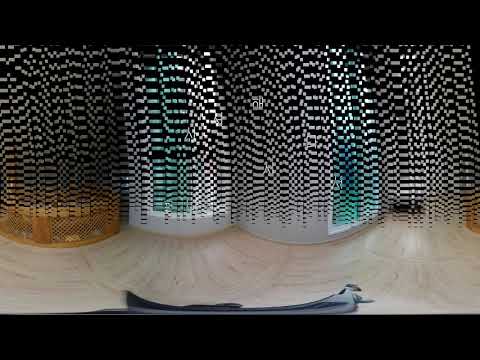The image is a computer-generated artwork showcasing four cylindrical architectural designs set against a horizontally aligned rectangular frame with thick black borders at the top and bottom. The lower part of the image features a marbled tile or countertop surface in shades of white and light gray. Partially visible on the countertop is an indiscernible silver or gray object.

Centered in the composition, the four cylindrical structures display varying colors and patterns. The leftmost cylinder has a rust-colored base transitioning into a silver and black upper section with white windows or docks. Adjacent to it, the second cylinder sports a light gray base accented with a middle section tinged in green, and continues with the silver and black theme towards the top. The third cylinder, similar in pattern to the second, is larger and also features a light gray base. The rightmost cylinder combines black at its base with additional rust color, maintaining a uniform silver and black finish upwards.

The overall setting of the image appears indoors, enhanced by the digital manipulation of the cylindrical designs, providing an abstract and artistic feel without any text. The color palette integrates black, gray, light gray, rust, turquoise, and green, contributing to the unique and captivating visual.